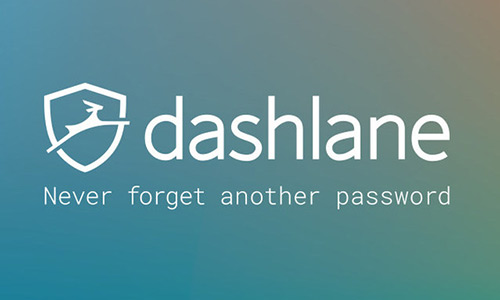The image features a simplistic yet carefully designed logo for Dashlane. At the center, the brand name "dashlane" is displayed in all lowercase letters, employing a clean and modern font. Directly beneath the brand name, the tagline "never forget another password" is presented in a slightly smaller text size. Notably, the article "in" within the tagline is capitalized, which stands out due to the sentence case used in the rest of the tagline. The text exhibits a gradient effect, starting with a vibrant turquoise on the left and subtly transitioning through brownish-red to green towards the right.

To the left of the text, there is an emblem depicting a leaping deer enclosed within a badge. The deer, in a dynamic pose, aptly symbolizes swiftness and agility, resonating with the brand name "Dashlane." The entire logo, including text and the deer emblem, is rendered in white, standing out against the background.

The overall aesthetic hints at a digital design, possibly suggesting the logo's application in a variety of digital platforms, though no specific device context such as a timestamp implies it is used on a laptop or smartphone is discernible. The lack of additional identifying features gives the impression of a straightforward copy-and-paste job.